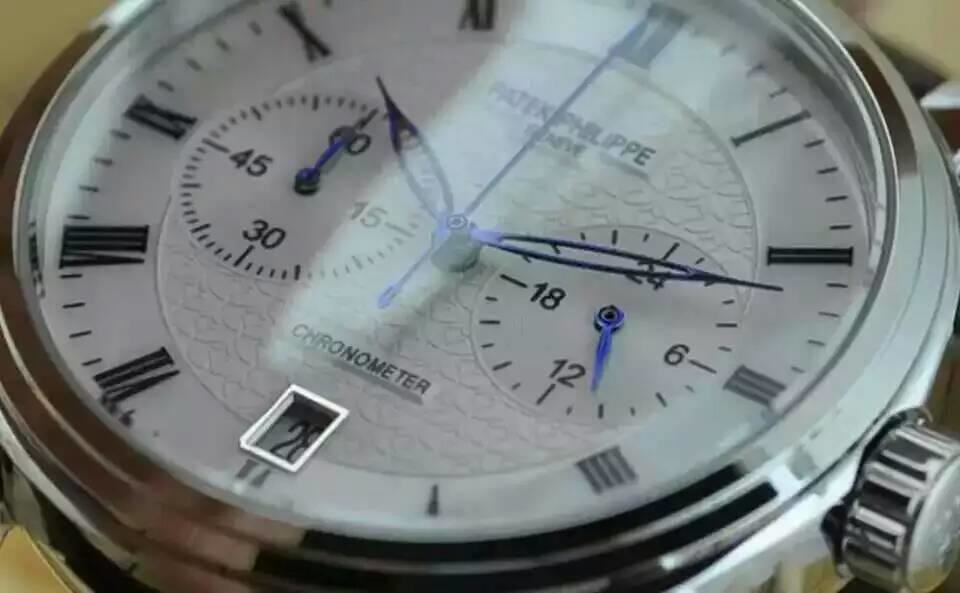This close-up photograph captures the intricate details of an exquisite Patek Philippe chronometer. Taken from a vertical standpoint, the image focuses on the watch's elegant face, completely omitting any view of the band. The timepiece features a pristine white dial encased in a refined silver bezel. The black Roman numerals stand out sharply against the white background, adding a touch of classic sophistication. Central to the face is a polished silver dial indicating the time, currently showing approximately 10:11. Additionally, two smaller sub-dials are visible, their functions not immediately apparent but contributing to the watch's complex and luxurious design.